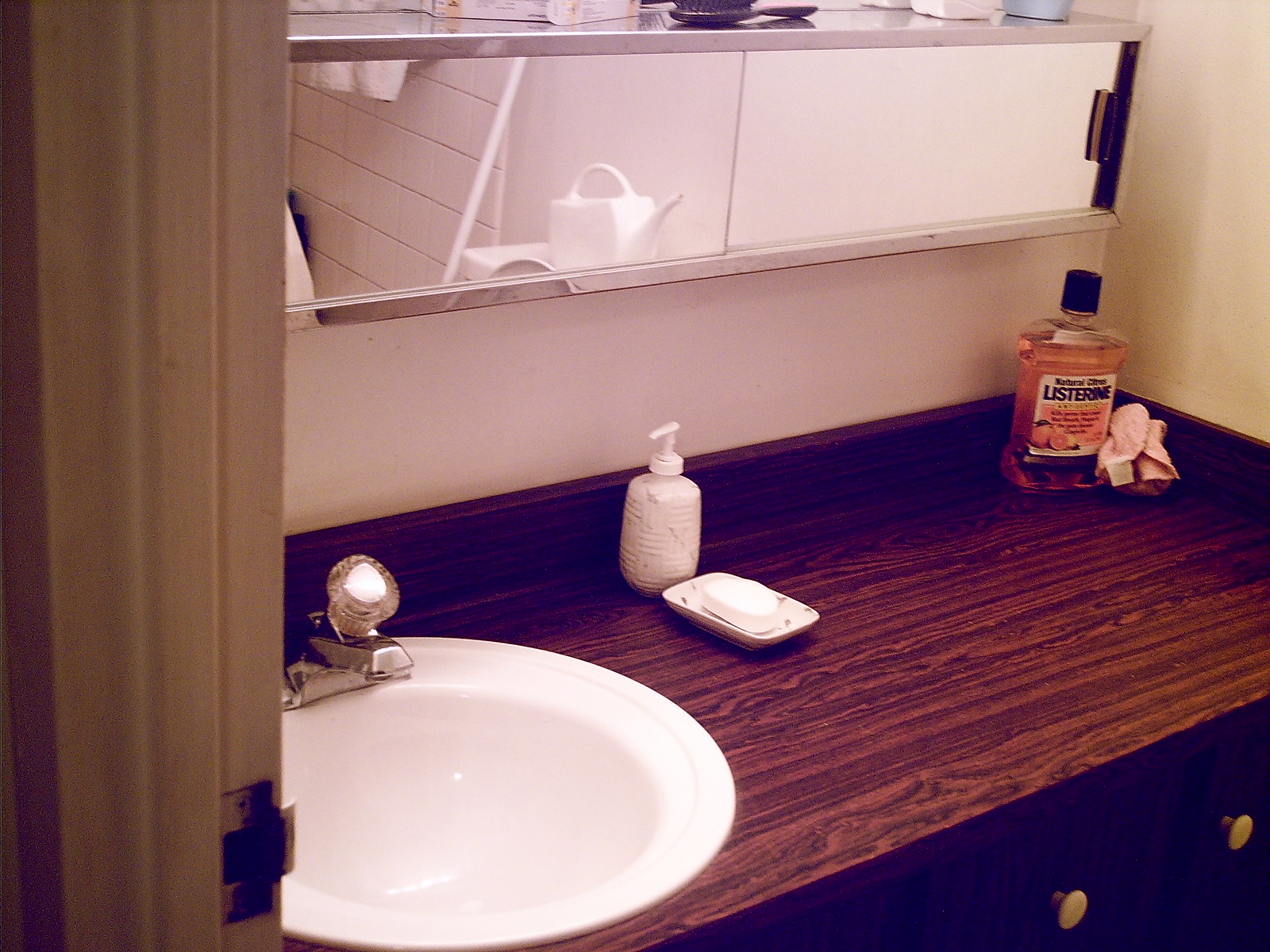In this photograph, the interior of a bathroom is captured with a soft, purple-tinted filter that adds a delicate hue to the scene. On the left side of the image, part of the door frame and the latch mechanism are visible, hinting at the entrance. The central focus of the image is a dark wooden countertop. In the lower right corner of the photo, two handles indicate the presence of cabinetry beneath the counter.

Prominently featured on the counter is a pristine white circular sink with a single faucet handle, designed to control water flow and temperature. To the left of the sink sits a soap dish containing a bar of soap and a pump dispenser. On the far right corner of the counter, an orange bottle of Listerine and a neatly folded rag are placed.

Above the countertop hangs a mirror reflecting more of the bathroom. In the mirror's reflection, part of the shower area and a toilet can be seen. A bottle rests atop the toilet, adding another layer of detail to the composition. This image provides a comprehensive and serene glimpse into a neatly arranged bathroom space.